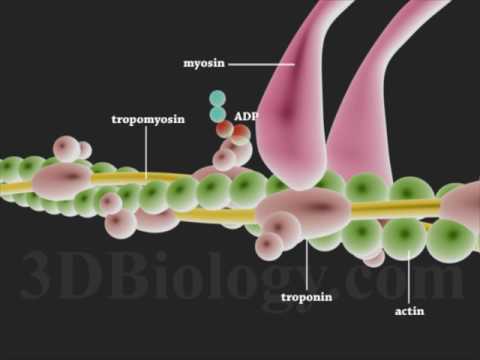This digital image from 3dbiology.com features a molecular diagram set against a black background with grey text prominently displaying the website name. The detailed illustration showcases the interplay of various proteins and molecules involved in muscle contraction. Myosin is depicted in pink, while tropomyosin is represented with green dots. ADP is marked with a combination of blue, red, and pink spots. Troponin is shown in pink, and actin appears as green elements. The diagram highlights how these components attach to muscle fibers, with yellow cords interlaced with green and pink dots, and additional pink structures descending from the top right. Arrows and labels point to each molecular component, emphasizing their roles and interactions.